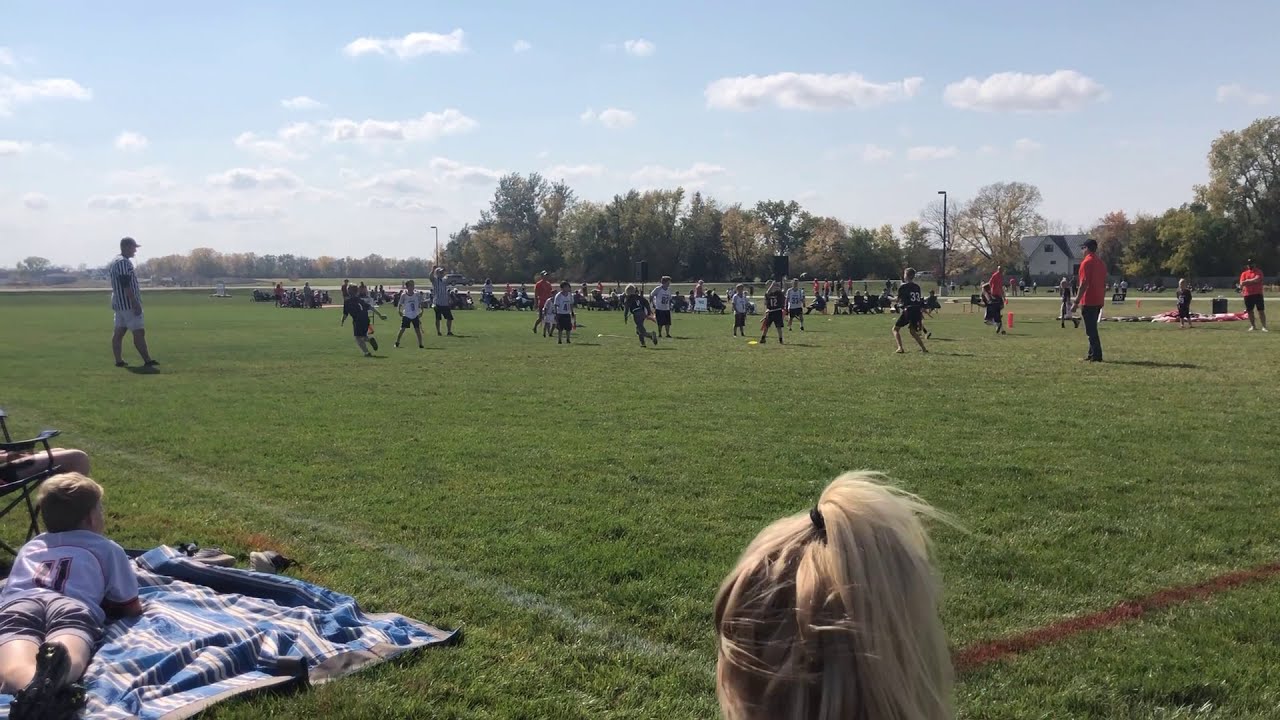The image showcases an outdoor sports field under a blue sky dotted with white clouds. In the foreground, to the left, a young boy with very blonde hair is lying on a blue and white striped blanket, watching the game. Nearby, there's a lawn chair positioned for spectators. Dominating the foreground, you can see the back of a woman’s head with light blonde hair tied up in a ponytail, also observing the game.

The main action unfolds in the middle distance where children are playing on a green grassy field. The game appears to be either soccer or a friendly match of football or Ultimate Frisbee, though no ball or goalposts are visible. The players are divided into two teams—one in black and the other in white and black shirts. Referees, coaches, and adults also dot the field, overseeing the youngsters who are in attentive, ready positions.

Beyond the field, the background consists of a row of trees and a distant house, underlining the serene, outdoor setting.